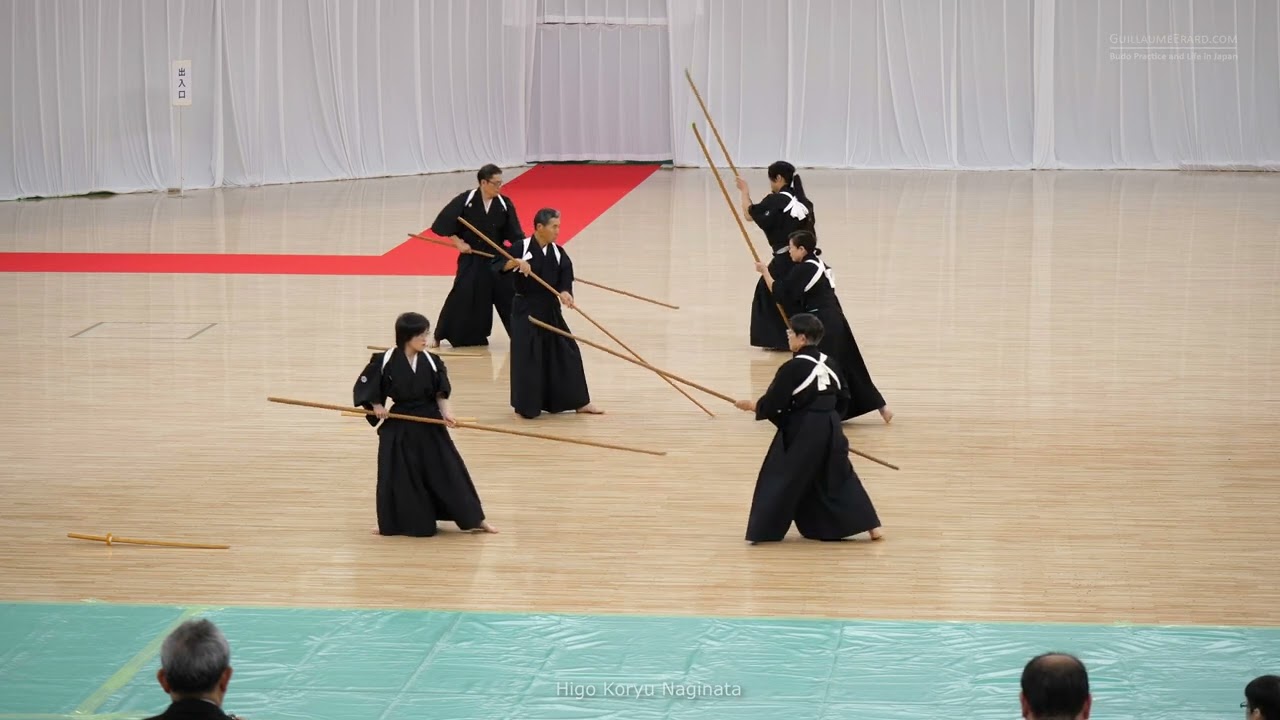The photograph captures an indoor martial arts demonstration taking place on a gymnasium floor with six practitioners engaged in combat techniques. Each person is dressed in black robes with distinctive white criss-cross patterns on the back, evoking a priest-like appearance. They each wield a long, skinny wooden pole, approximately 10 feet in length, resembling oversized dowel rods or chopsticks. These practitioners, a mixture of genders, appear to be paired off against each other. The room features light wood-colored flooring common to basketball courts, with a green plastic sheet protecting the floor in the foreground. A white curtain hangs in the background, accompanied by a red boundary line indicative of a basketball court and a red carpet running from the doorway. The bottom edge of the photograph includes the heads of three audience members, one on the left and two on the right. Text in the center along the bottom edge reads "Naginata," indicating the martial art being demonstrated.